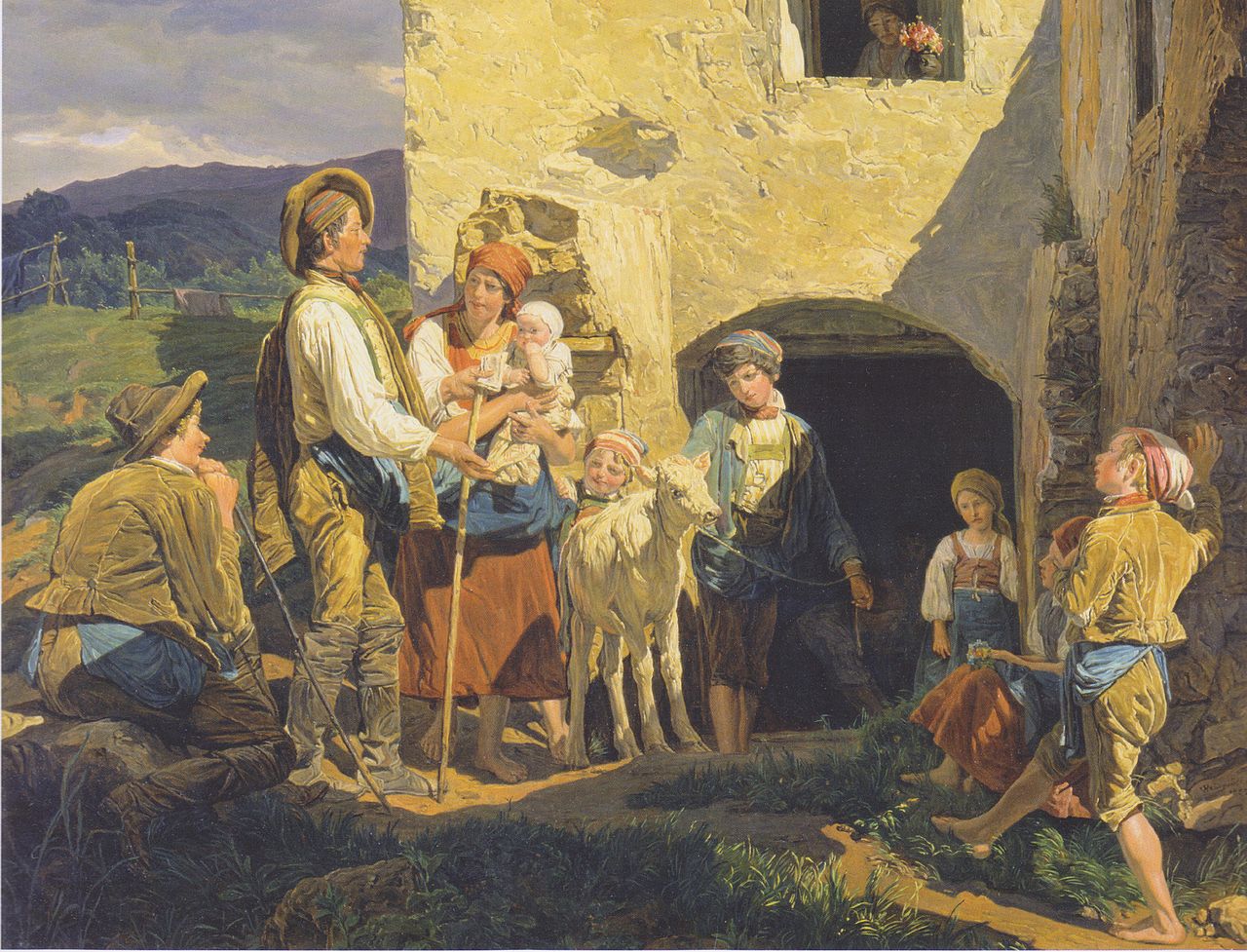The painting depicts a pastoral scene set against a backdrop of verdant rolling hills and towering blue-gray mountains. In the foreground, a family has gathered outside a building that resembles an old western castle with a yellowish-beige stucco wall and a giant doorway. The scene is animated by the presence of various family members engaged in different activities.

A central figure, a man in rugged brown pants and knee-high boots, stands in the midst of the group holding a staff. His attire includes a billowy white shirt and an intricately wrapped cap of red, blue, and brown fabric. He seems to be engaged in conversation with a woman donning a long red dress, white sleeves, a blue apron, and a red scarf. She is holding an infant dressed in white, while standing next to a young boy in a blue jacket, short brown pants, and a red and blue cap, who is holding a white calf by a rope.

To the right of the group, another person in a green jacket sits barefoot on the grass, their feet outstretched and a green hat lying beside them. A young boy peeks from behind the calf, wearing a red, blue, and white cap, suggesting a familial connection. Nearby, another individual is seen holding onto a wall, while a child peers from a window adorned with a pink plant.

The image has a timeless quality, evoking a sense of rustic charm and familial bond set against a natural backdrop of lush grass and distant mountains. The intricate clothing details, such as the woman's brown headdress and the man's knee-high boots, enhance the historical ambiance of the scene.